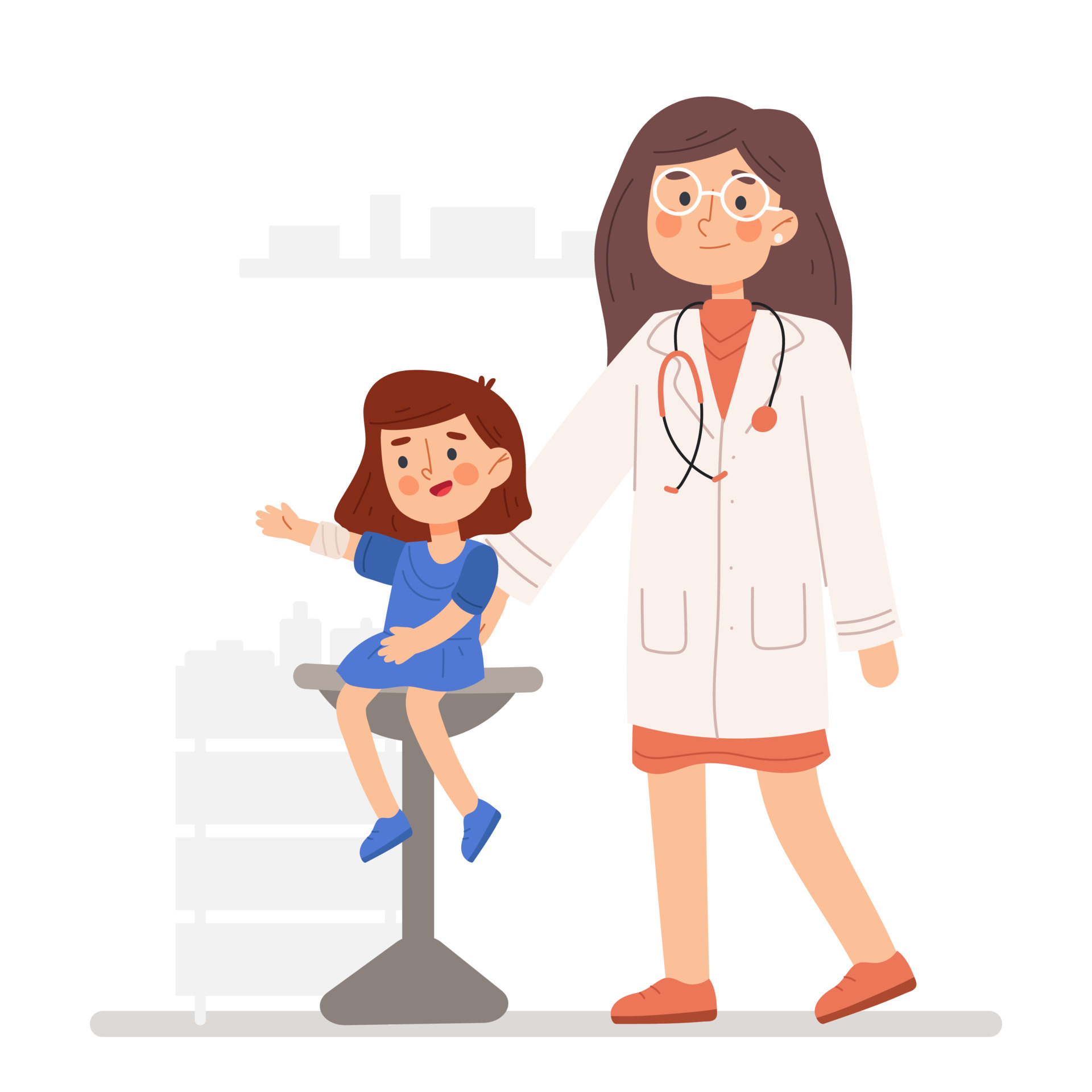In this colorful and cheerful cartoon-style illustration, a female doctor with brown hair, white-rimmed glasses, and rosy cheeks is depicted wearing a white medical coat over a dress, accessorized with a stethoscope around her neck and brown shoes. She is sitting on a metal stool in what appears to be a doctor's office, with a blurred white background indicating the environment. To her left, a young girl with brown hair and rosy cheeks, dressed in a blue dress and blue shoes, sits on a large gray seat. The girl's arm is bandaged, possibly indicating it has been treated or she has received a vaccine. Both characters exhibit a friendly and happy demeanor, accentuated by the smooth-edged, vibrant, and distinctive cartoon style that adds a sense of joyfulness to the scene.